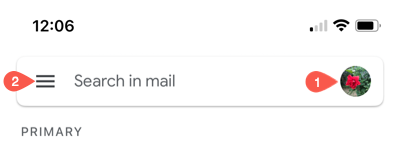An image captured at 12:06, indicated by the timestamp in the top left corner, exhibits a typical smartphone screen. In the top right corner, the screen shows a Wi-Fi indicator with one out of four bars, a black Wi-Fi symbol, and a battery icon that appears to be approximately 78-79% charged, equating to about three-fourths full.

Below these icons, a search field is displayed labeled 'Search in Mail.' Within this search field, there are three black lines accompanied by an orange sideways teardrop-shaped icon on their left, containing the number '2' inside. Adjacent to this, on the right, there is a profile picture depicting a green bush adorned with a pink flower. This image also features a similar sideways teardrop-shaped icon with the number '1' in white.

Beneath this section, the word 'Primary' is displayed in gray letters. The rest of the screen is a plain white background, offering no additional visible content or context.